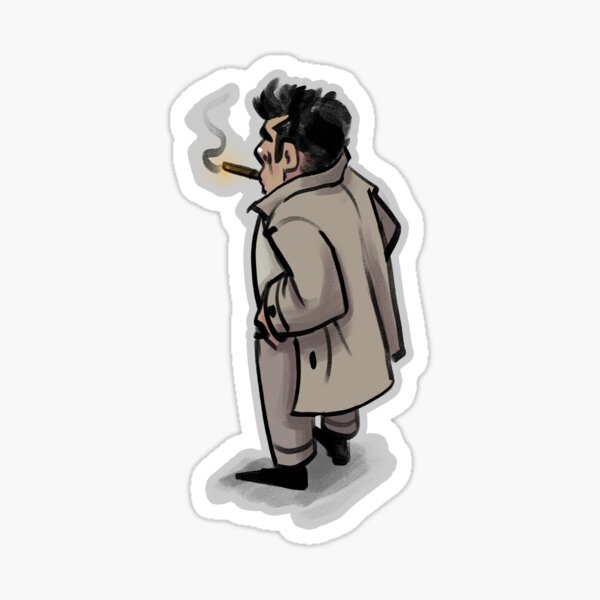The image depicts a cartoon drawing of a rugged man, reminiscent of a detective, primarily seen from behind and slightly turned to his side, facing left. He is wearing a grayish-brown trench coat, which is unbuttoned to reveal a lighter brown shirt beneath. The trench coat also features what appear to be button-like marks on the sleeve and body. His hands are tucked into his pockets, and he's dressed in matching brown trousers and black pointy shoes. He has high, dark black hair and bushy eyebrows, holding a lit cigar from which a trail of smoke arises. The background is predominantly white, surrounded by a gradient of light gray, giving it a sticker-like appearance against the stark white.